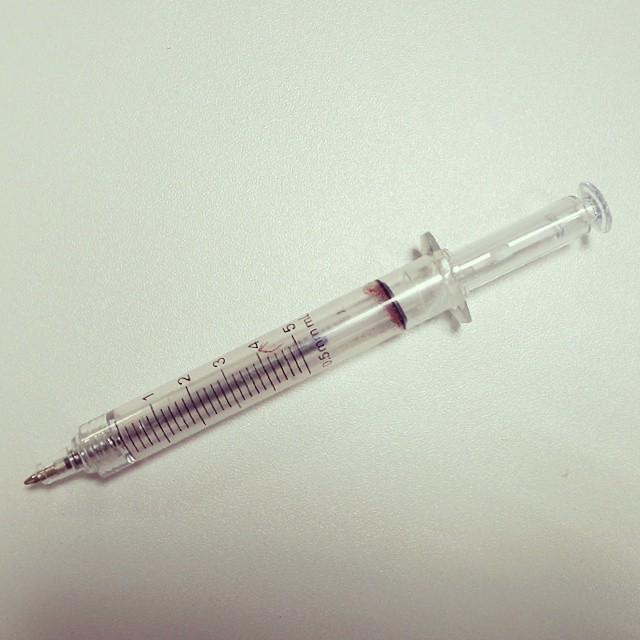The image is a vertical rectangular photograph of an ink pen designed to look like a syringe. It rests diagonally from the lower left to the upper right on a textured grayish-white background, which darkens toward the bottom. The pen, crafted from clear plastic, mimics a medical syringe with its cylindrical body and plunger. The clear main body of the pen is marked with black gradations from 0 to 5, and the bottom is labeled with "0.5 milliliter." Inside the clear tubing, black ink is visible, resembling the fluid inside a real syringe. The plunger, also clear, is fitted with a black gasket area near the base and features a small stop to allow full compression.